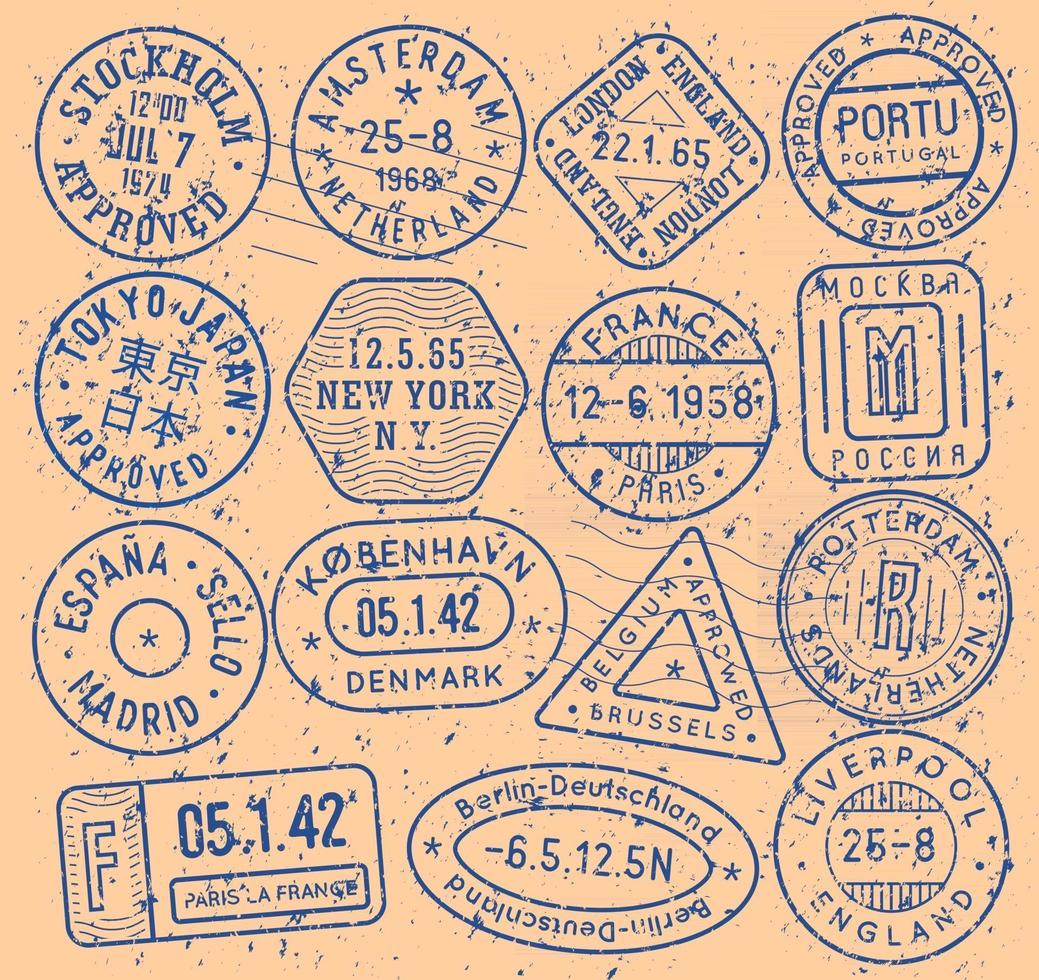The image is a poster showcasing a collection of postal stamps from different countries, set against a light tan background. The stamps, primarily blue in color, resemble the kind you would find in a passport and feature a variety of shapes including circles, a triangle, an octagon, a rectangle, and an oval. At the top, there is a stamp from Stockholm, Sweden, dated July 7th, 1974 with an "Approved" mark. Next to it is a stamp from Amsterdam, The Netherlands, dated 25 August 1968. Other notable stamps include ones from London, England, Portugal, Tokyo, Japan, New York City, USA, and various locations in France such as Paris and Macbeth. Additional stamps represent Madrid, Spain; Copenhagen, Denmark; Brussels, Belgium; Rotterdam, The Netherlands; Berlin, Germany; and Liverpool, England. The detailed stamps give a sense of international travel and history, each marked with unique details and securing its place on the poster.